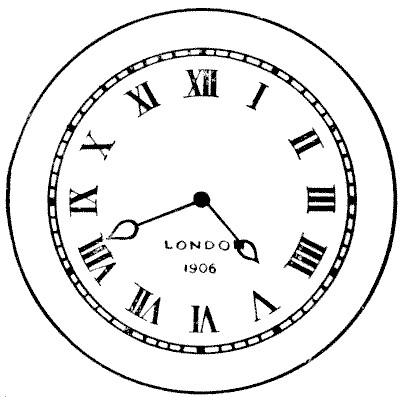This is a highly detailed, simple black-and-white line drawing of an old-fashioned analog clock. The clock is circular, featuring an outer and an inner circle with alternating black and white stripes. The clock face is marked with black Roman numerals arranged in the standard 1-12 positions, with minute tick marks between them; the larger, darker lines denote the hours. At the bottom of the clock face, it is labeled "London, 1906." A small black dot marks the center of the clock where the two black hands—styled with straight lines and ending in teardrop or leaf shapes—indicate the time as approximately 3:40. The image is devoid of any additional ornamentation, emphasizing the clock's vintage design.